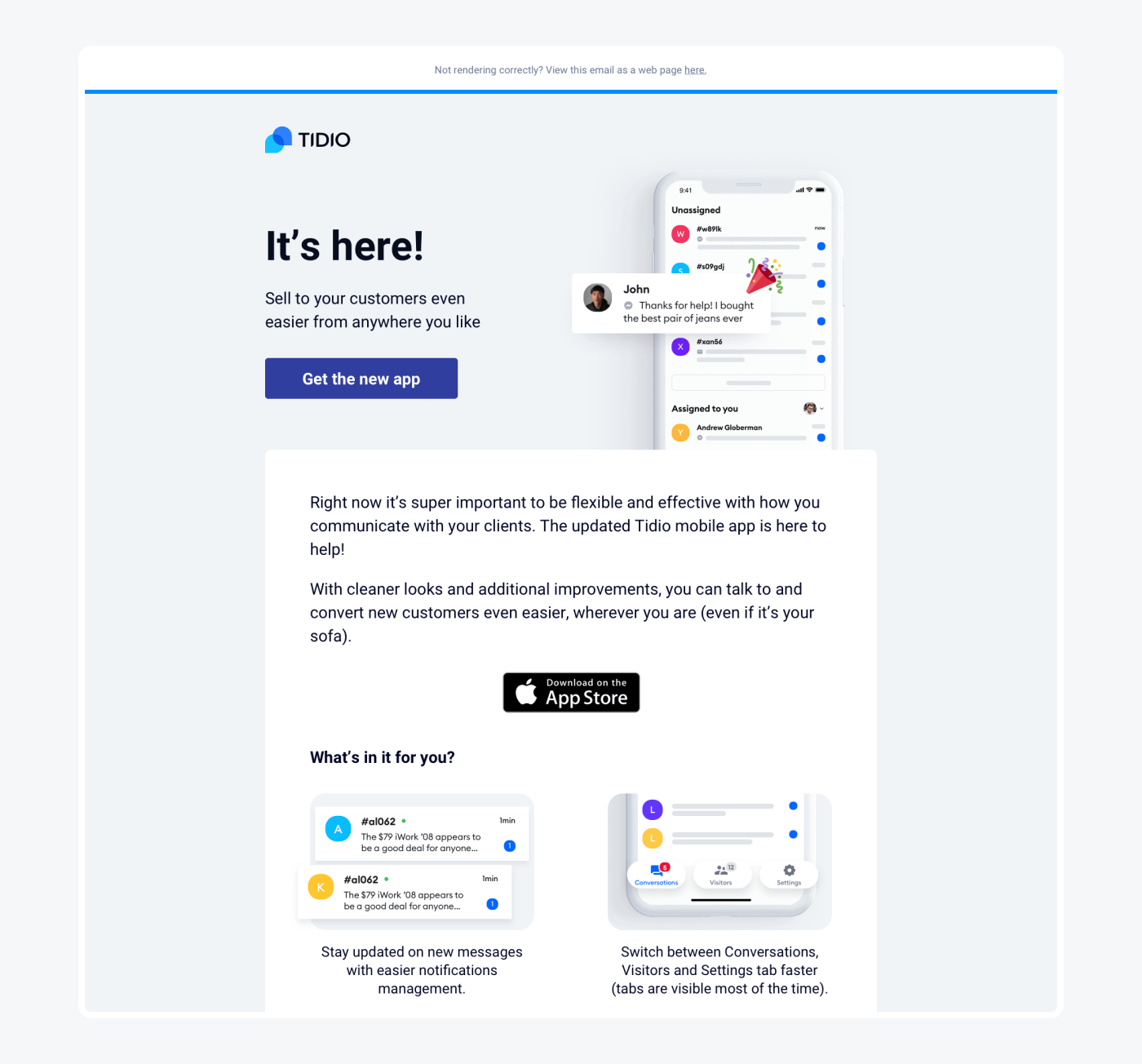A detailed descriptive caption for the image:

"This is a promotional webpage for TIDIO, displaying their updated mobile app designed for client communication management. The TIDIO logo, featuring two overlapping communication balloons in different shades of blue, is prominently displayed. The page highlights the app's availability on the Apple App Store, as evidenced by a visible App Store badge. The updated app promises enhanced notification management, allowing users to stay updated on messages from clients more effectively. The app also supports seamless switching between conversations, positioning itself as a specialized tool for client communications rather than personal messaging. The background is a light bluish gray with a large white block containing black text. Scattered across the page are multiple screenshots and graphics showcasing the app’s interface and features."